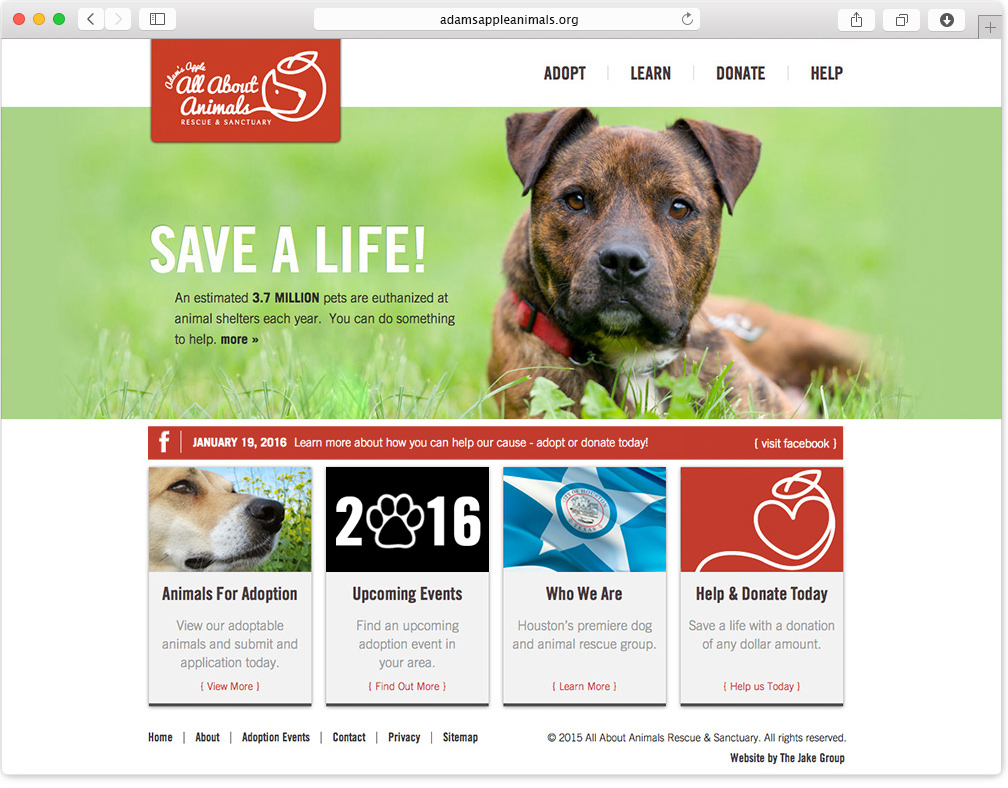This is a comprehensive screenshot of the Adams Apple Animals website. At the top of the page, there's a sleek gray navigation bar. On the right side of the bar, there's a plus sign enclosed in a box. To its left are three white buttons: the first one features a gray circle with a white downward arrow, the second shows two overlapping squares, and the third displays a square with an upward arrow. Centered within the gray bar is the website URL: AdamsAppleAnimals.org. Toward the left of the bar, three colored dots—red, yellow, and orange—are lined up.

Directly below the gray navigation bar, there is a white menu bar with clickable links labeled Adopt, Learn, Donate, and Help, providing quick access to different sections of the site.

In the top-left corner of the webpage, there's a distinctive red rectangle featuring the site’s logo in elegant white cursive font: "All About Animals." Notably, the "S" in "Animals" stylishly extends into a circular design encompassing a cartoon dog’s head. Beneath the logo, the text "Rescue and Sanctuary" is displayed.

Dominating the main content area is an adorable photograph of a mixed-breed dog, possibly a pit bull-terrier mix, with a brindle coat. The dog, with its black nose and brown eyes, exudes cuteness as it rests in a lush green field, gazing forward attentively.